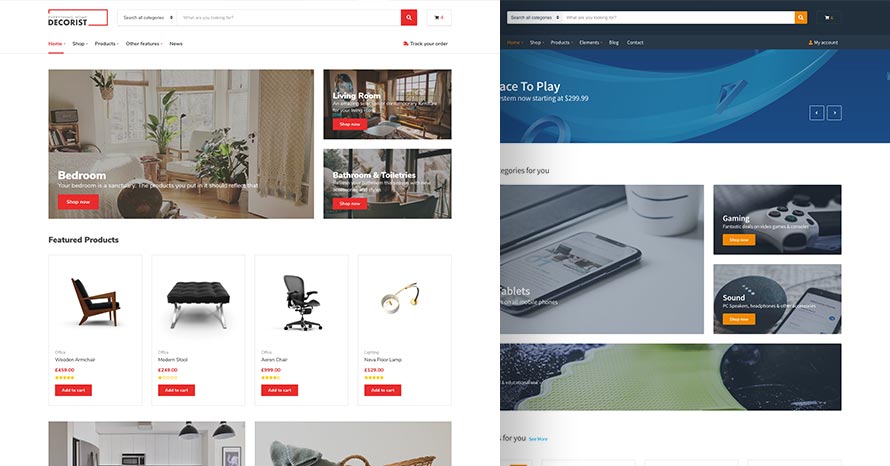The image consists of two side-by-side screenshots showcasing different sections of two websites.

**Left Screenshot:**
The website on the left is identified as Decorist, with a recognizable logo situated in the upper left-hand corner against a rectangular background. Adjacent to the logo is a menu which is not clearly legible, followed by a search field featuring a red button. Beneath this is a main menu bar with "Home" and "Shop" options, though the subsequent text is too small to discern. The central part of the page prominently displays an image of an interior bedroom with a semi-transparent overlay and the text "Bedroom Shop Now" to the right. Below this, there are two stacked images labeled "Living Room" and "Bathroom & Toiletries," each accompanied by "Shop Now" options. Lower on the page, there are product images against white backgrounds, including a chair, a stool, an office chair resembling the quality of an Aeron chair, and a lamp. Although the titles and prices are not readable, red "Add to Cart" buttons are visible below each product. Additionally, there are two more partially cut-off photos at the bottom.

**Right Screenshot:**
The right screenshot depicts another website with a layout similar to Decorist's. The header features a blue graphic, a search bar, and an unspecified menu. The page showcases a grid of photos: one on the left featuring a phone on a desk, followed by images labeled "Gaming" and "Sound." The exact details of the remaining sections are unclear due to the small size and illegibility of the text.

Overall, these screenshots illustrate different e-commerce platforms with visually engaging layouts focused on home decor and electronic gadgets, respectively.